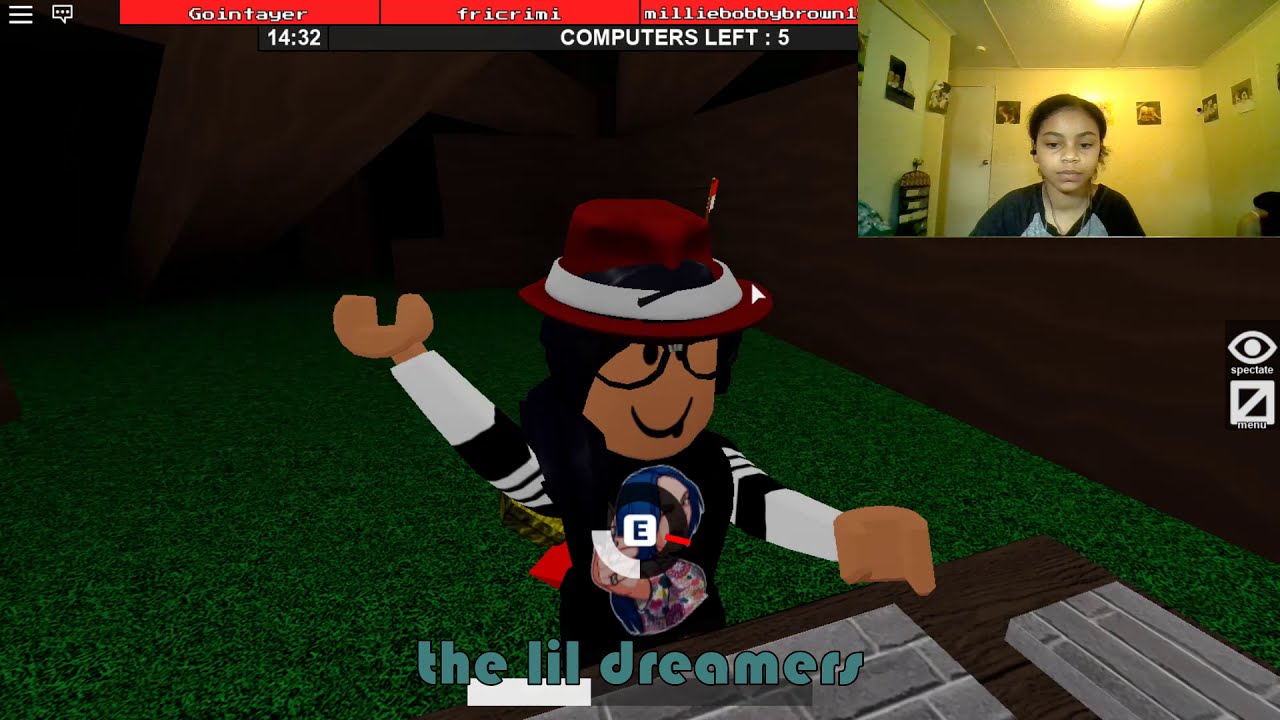In this detailed screenshot of a video game, we see a split-screen setup featuring a young girl playing the game in the top right corner and the game itself taking up the rest of the screen. The girl, who appears to be of African descent and around 12 years old, has her hair pulled back and is wearing a dark gray T-shirt, sitting in a bedroom with a yellowish glow. 

The game displayed shows a custom, cartoonish DJ character reminiscent of LEGO with a vibrant red hat similar to Michael Jackson's from the "Smooth Criminal" video, black glasses, and a T-shirt. The character is positioned on a grassroots platform, with the left hand on a turntable and the right hand raised in the air. The wooden table with grey bricks is part of the setting, indicating a paused or stationary scene.

The top of the gaming screen has a red navigation bar with the labels "Go in TAYER" and "Creamy" or possibly "F-R-I-C-I-M-I," suggesting these are menu items or teammates. Below, a black bar displays “Computers Left” with a timestamp reading 1432. At the bottom, green text with a black outline spells out "The Little Dreamers," which is the game's title or a significant in-game element.